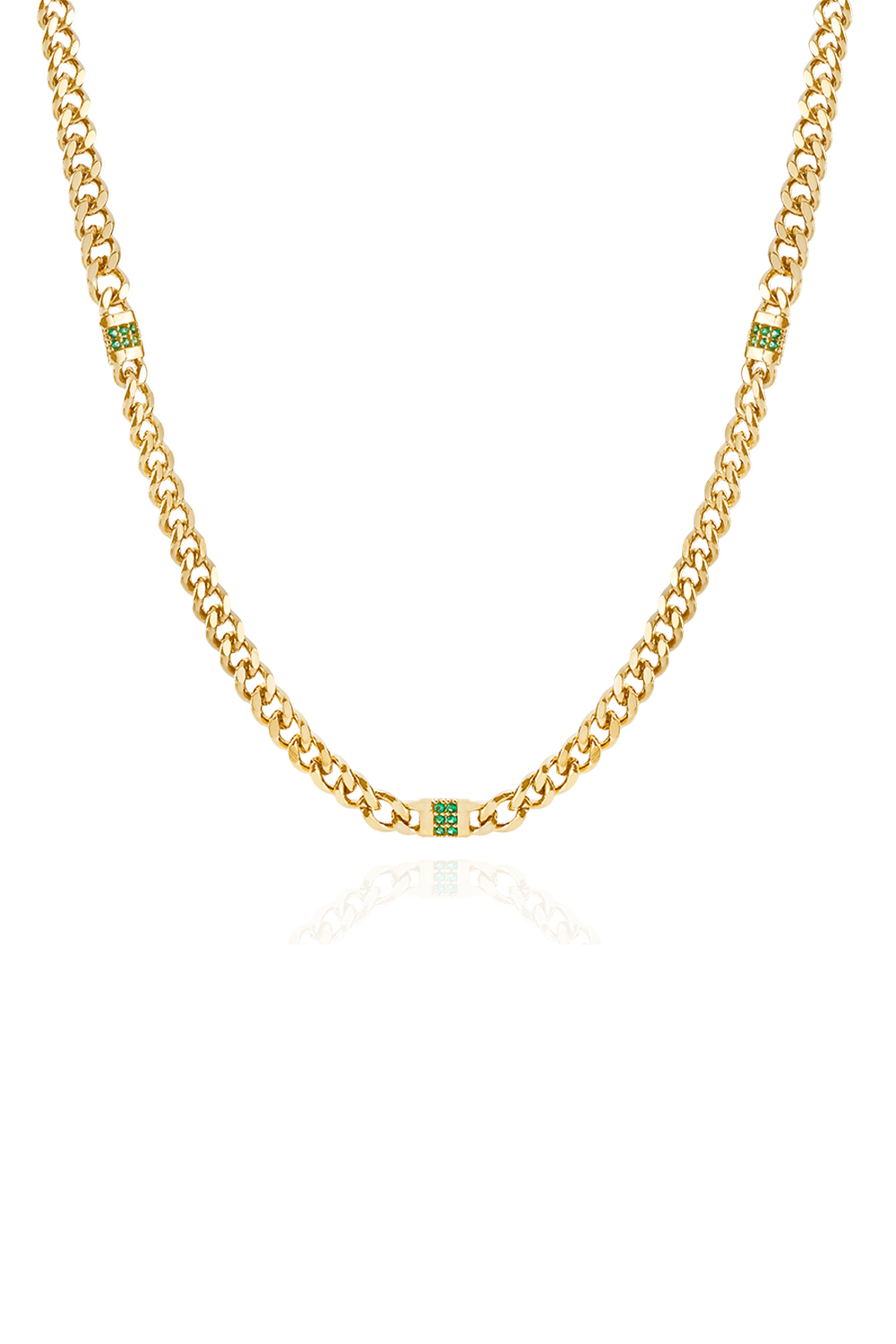This is a full-color photograph of a decorative gold chain necklace set against a white background, giving the impression of it being superimposed. The necklace forms a U-shape, partially displayed with neither clasps nor ends visible at the top. The chain features decorative embellishments, specifically clusters of small green stones distributed across its length. Notably, three sections along the chain are adorned with green stones: halfway up the left side, halfway up the right side, and towards the bottom. The bottom section distinctively has a pendant-like square arrangement formed by six tiny green stones. The chain's reflection is subtly visible at the bottom. The image contains no text or branding.